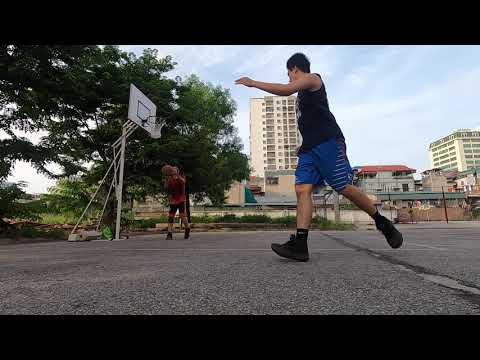The image depicts an urban basketball court with a cement surface, set against the backdrop of a cityscape with skyscrapers and various buildings. The court features a basketball hoop on a white pole located on the left side. Dominating the foreground, a Caucasian man is caught in motion, running by with one arm up, his right foot forward and left leg behind as if he’s turning and running. He is wearing light blue shorts with a design on the side, dark socks, dark tennis shoes, and a dark tank top. He has short dark hair, and his face is partially obscured from view. In the background, another man is positioned under the hoop, poised to throw the basketball. He's wearing a red shirt, dark shorts, dark shoes, and a black knee support. This man’s figure is partially obscured by distance and his action pose. Surrounding the court are tall green trees and bushes. Beyond the trees, the skyline consists of several tall apartment buildings and other structures, including one shorter building with a red roof. In the far distance, the light blue sky is dotted with faint clouds.